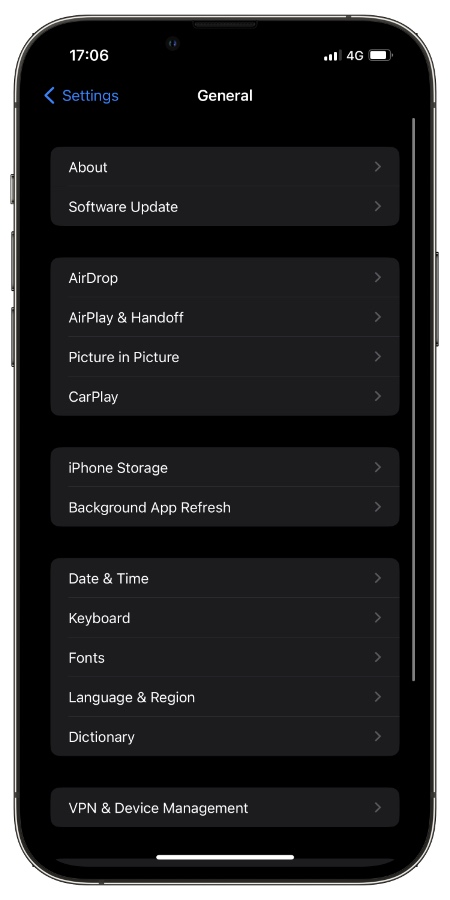The image depicts a close-up screenshot of a cell phone displaying its Settings app. At the top of the screen, the word "Settings" appears in blue text accompanied by a left-pointing arrow. 

Below, the "General" section is prominently listed, with subcategories including "About" and "Software Update." A black dividing line separates this section from the next, which contains four options within their own rectangle: "AirDrop," "AirPlay & Handoff," "Picture in Picture," and "CarPlay." Each option is accompanied by a right-pointing arrow, indicating further options or submenus.

Further down, another black dividing line separates the "iPhone Storage" and "Background App Refresh" settings, each also within a rectangle with right-pointing arrows. 

The next section, also divided by a black line, includes five settings: "Date & Time," "Keyboard," "Fonts," "Language & Region," and "Dictionary," each with a right-pointing arrow. 

The final setting, "VPN & Device Management," stands alone at the bottom, following another black dividing line and also features a right-pointing arrow.

The layout and icons clearly organize the variety of options available for tweaking the phone’s settings.